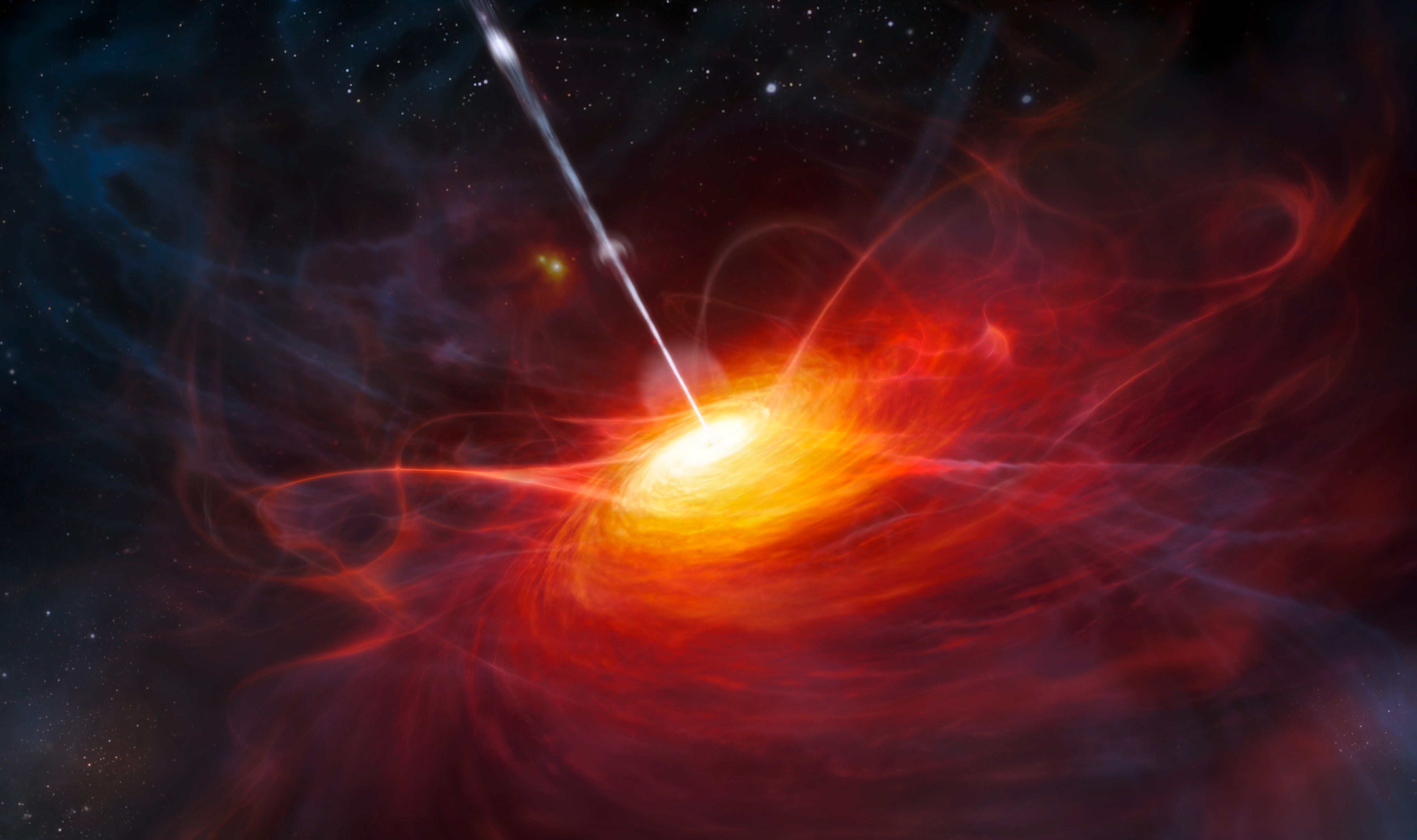Amidst a dark, star-dotted expanse suggestive of outer space, a mesmerizing, tornado-like vortex occupies the center of this rectangular landscape image. This dynamic, swirling formation is a blend of vibrant red and pink outer layers, transitioning smoothly to brilliant yellows and oranges as it spirals inward. At its core, a radiant white center emits a strong pillar of light that streaks vertically up through the image, cutting through the cosmos like a sunbeam. The vortex, webbed with intricate windy textures, gives an impression of fluid motion and energy, as if capturing a moment of astronomical significance in a contemporary, abstract style. The interplay of swirling colors and the bright central beam enhances the sense of movement and action within this captivating space-like scene.